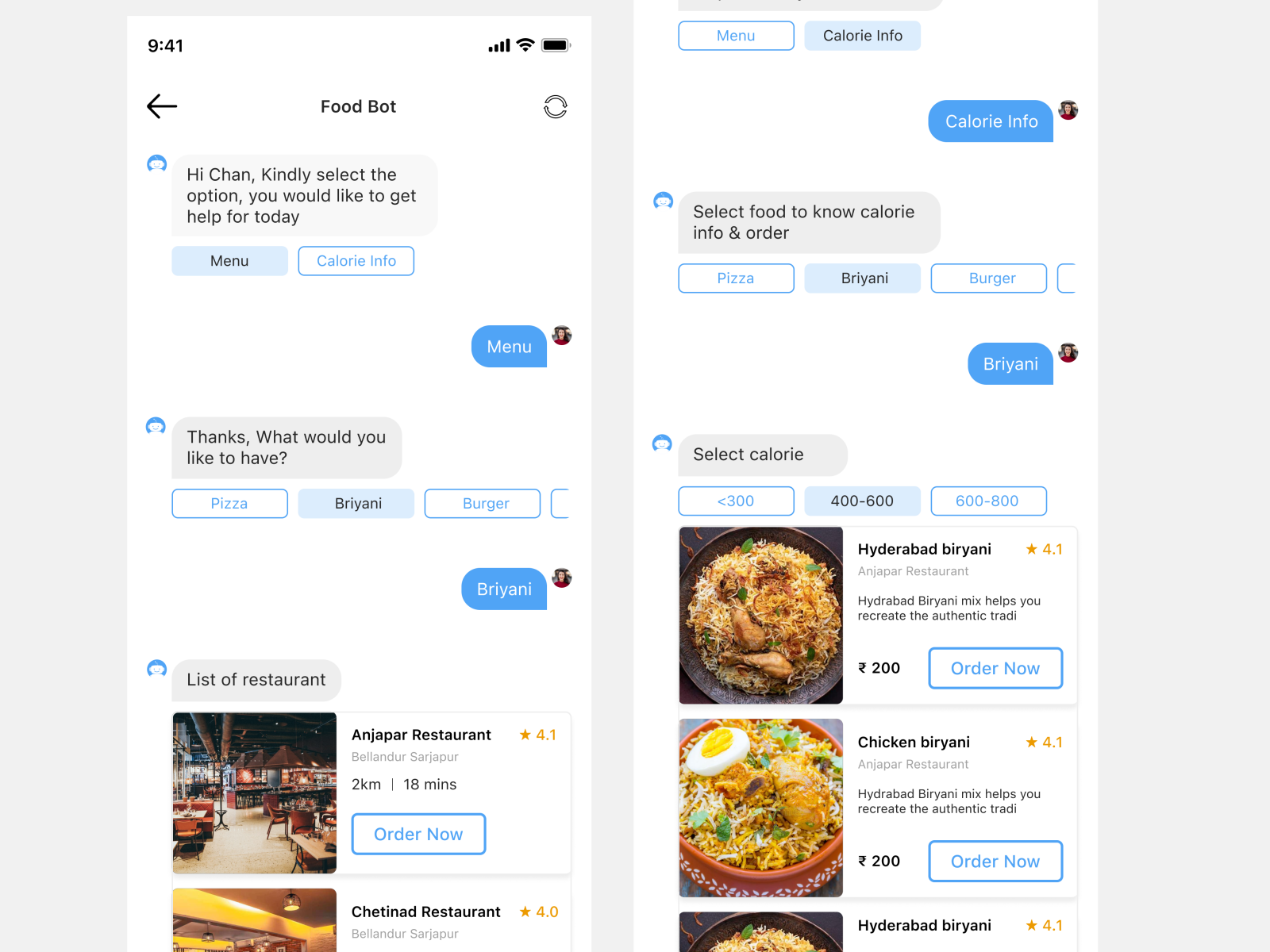Caption: 

This image portrays an interaction between a customer and a food bot, displayed across two vertical rectangular screens on a user's smartphone. 

On the first screen:
- The top-left corner shows the time "9:41" in black text, with a full battery icon and five signal bars to the right.
- Below that, centrally positioned in black text, is the title "Food Bot".
- The food bot initiates the conversation with a gray text bubble saying, "Hi Chan, kindly select the option you would like to get help for today."
- The user, Chan, responds with "Menu" in a bright blue text bubble, accompanied by his profile picture.
- The food bot replies in a gray text bubble, "Thanks, what would you like to have?" 
- Chan answers "Biryani", followed by the food bot displaying "List of restaurants" and a vertical list of restaurant options beneath it.

On the second screen:
- Chan requests "Calorie info" in another bright blue text bubble.
- The food bot responds with, "Select food to know calorie info and order."
- Chan again specifies "Biryani".
- The food bot presents calorie information for various dishes, each with a white "Order Now" button featuring a bright blue border and text.

This comprehensive interaction demonstrates the food bot's functionality, guiding the user through menu selections, dietary information, and ordering options seamlessly.